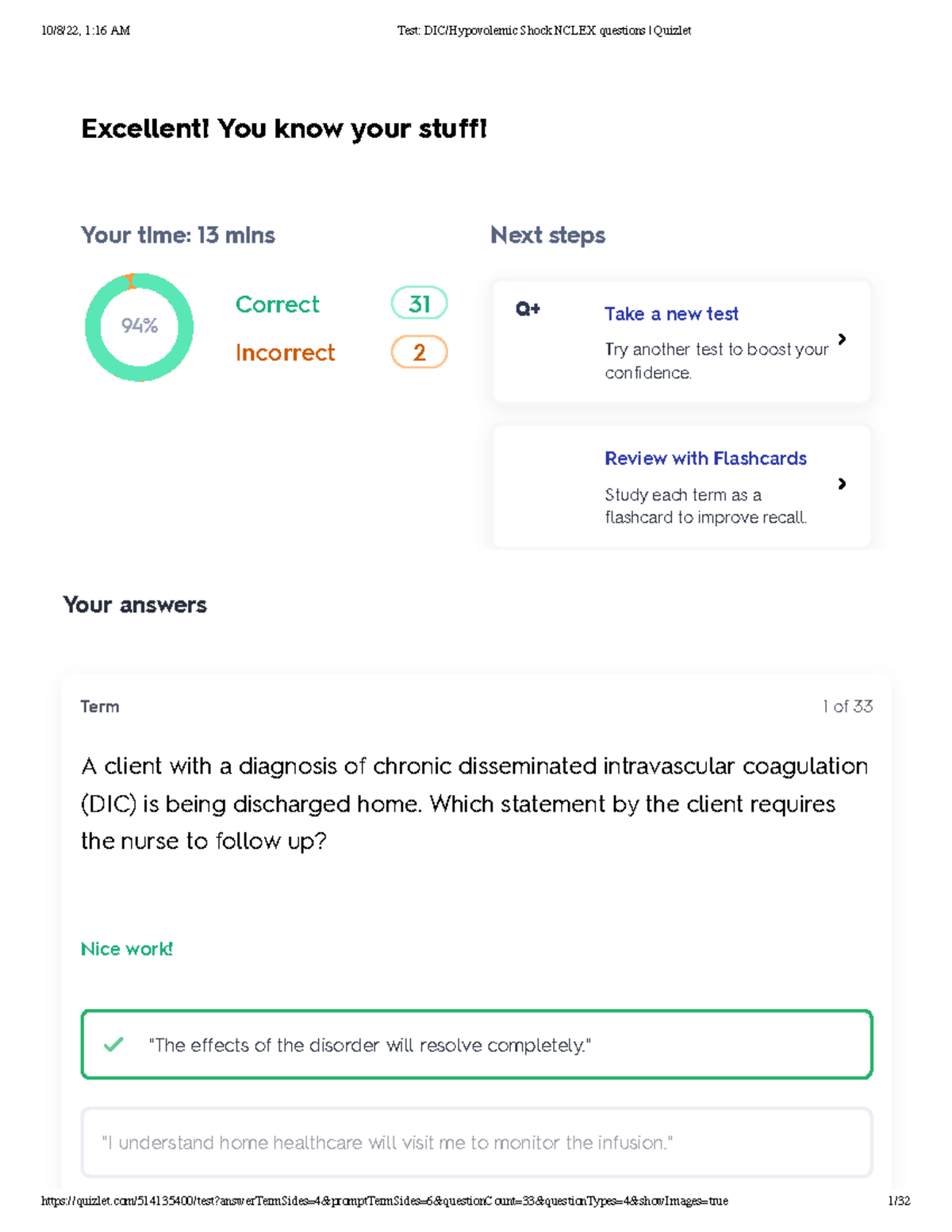This screenshot depicts a Quizlet test results page focused on NCLEX questions related to DIC (Disseminated Intravascular Coagulation) and hypovolemic shock, captured at 10:22:16 a.m. The test score is presented prominently with a green circular progress indicator displaying 94%, including a smaller orange section representing the incorrect answers. The user answered 31 questions correctly and 2 incorrectly, taking 13 minutes to complete the test. 

Several post-test options are available: taking a new test, trying another test for confidence building, and reviewing flashcards. These options are designed to enhance the user's understanding and recall. The detailed question review section begins with the first term of 33: "A client with a diagnosis of chronic disseminated intravascular coagulation (DIC) is being discharged home. Which statement by the client requires the nurse to follow up?" The correct answer, marked with a green checkmark, is "The effects of the disorder will resolve completely," which is flagged for follow-up because it indicates a possible misunderstanding by the patient.

Additional navigational details include pagination at the bottom right corner ("1/32") and a URL at the bottom left corner, leading to the specific Quizlet page where the test can be taken or reviewed.